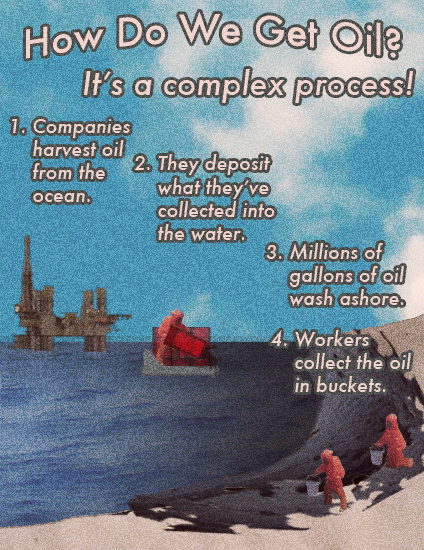The image is an illustrated poster styled like an old-timey magazine cover. It prominently features the title "How do we get oil? It's a complex process!" in white text with a gray outline, set against a blue sky with white clouds. Below the title, a series of four steps is arranged in a curved arch from the top left to the bottom right:

1. Companies harvest oil from the ocean.
2. They deposit what they've collected into the water.
3. Millions of gallons of oil wash ashore.
4. Workers collect the oil in buckets.

The lower half of the poster includes detailed illustrations. On the center left, an oil rig stands tall, surrounded by ocean water. To the right, closer to the bottom, two men dressed in red hazmat suits (also described as orange in some accounts) with silver buckets walk along a beach stained with oil. The visual narrative captures the process of oil extraction and its environmental impact vividly.